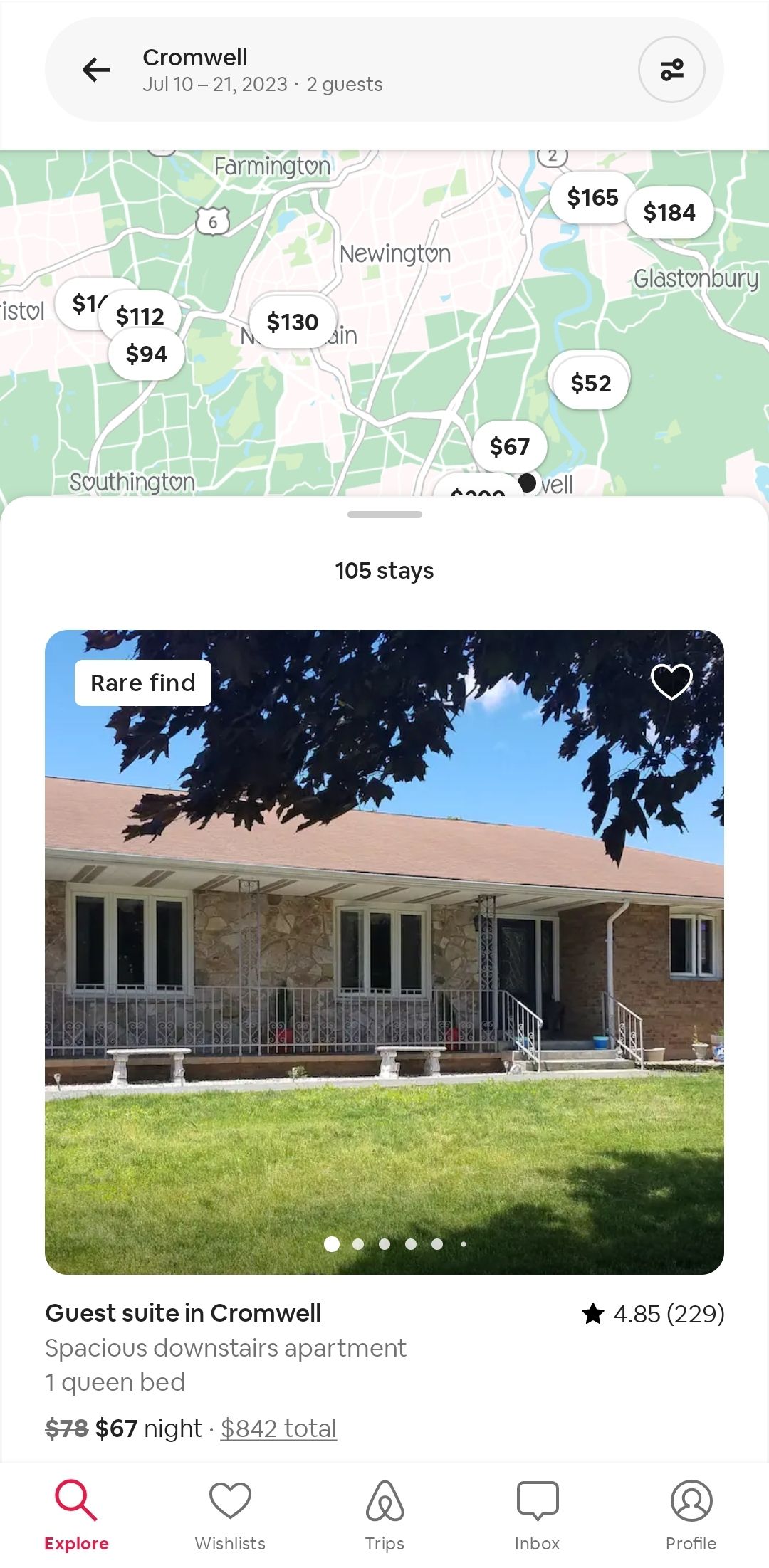At the top of the image is a white box with black text that reads "Cromwell July JUL 10th to 21st 2023," followed by "two guests." To the left of this text is a black back arrow, and on the right are two black bar icons inside a circle. 

Below this is a map displaying various shades of green and off-white, dotted with white bubbles showing black prices such as $1.12, $94, $130, $67, $52, $165, and $184. The map also includes city names like Farmington, Newton, Glastonbury, and Southington.

Further down is a gray bar with black text that reads "105 stays." This is followed by an image of a business with a description in a white and black box: "we're fine," accompanied by a white heart icon. The business features a stacked stone exterior in shades of light tan and gray, reminiscent of a 1960s design. It has white windows, a slightly pinkish-brown roof, some wrought iron elements, stone benches outside, green grass, and a blue sky.

At the bottom of the image are a series of white dots and text in black that reads "guest suite and Cromwell spacious downstairs permit one queen bed." The price is listed as "$78" with a slash through it, followed by "$67 a night," amounting to "$842 total." Additionally, it boasts a "4.85 stars" rating from "229 reviews."

Finally, there are several icons at the very bottom: a pink magnifying glass labeled "explore," a heart with the label "wish list," a triangle symbol labeled "trips," a text bubble icon labeled "inbox," and a cartoon person icon labeled "profile."